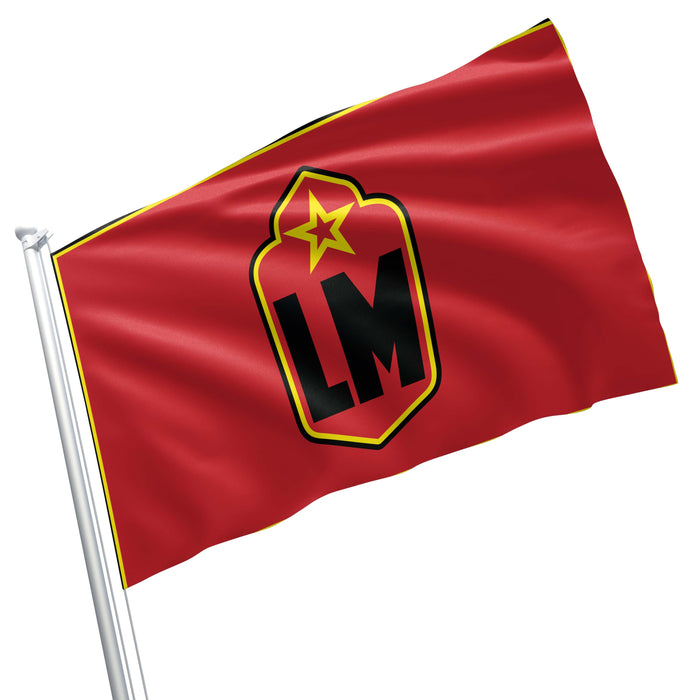This computer-generated image depicts a red flag on a white or possibly silver flagpole, set against a white or transparent background. The flag stretches diagonally from the bottom left to the top right corner of the frame. It features semi-rippled, fabric-like ridges for a realistic appearance. The flag is bordered with a black and yellow outline and prominently displays the bold letters "LM" in large black font. Above the letters, there's a yellow star with a red center. The emblem containing these elements is shield-shaped and intricately outlined. The flagpole's details are visible, including the string used to hoist the flag, adding to the overall realism of the image. The setup suggests simplicity, possibly indicating a design for a school or an organization.